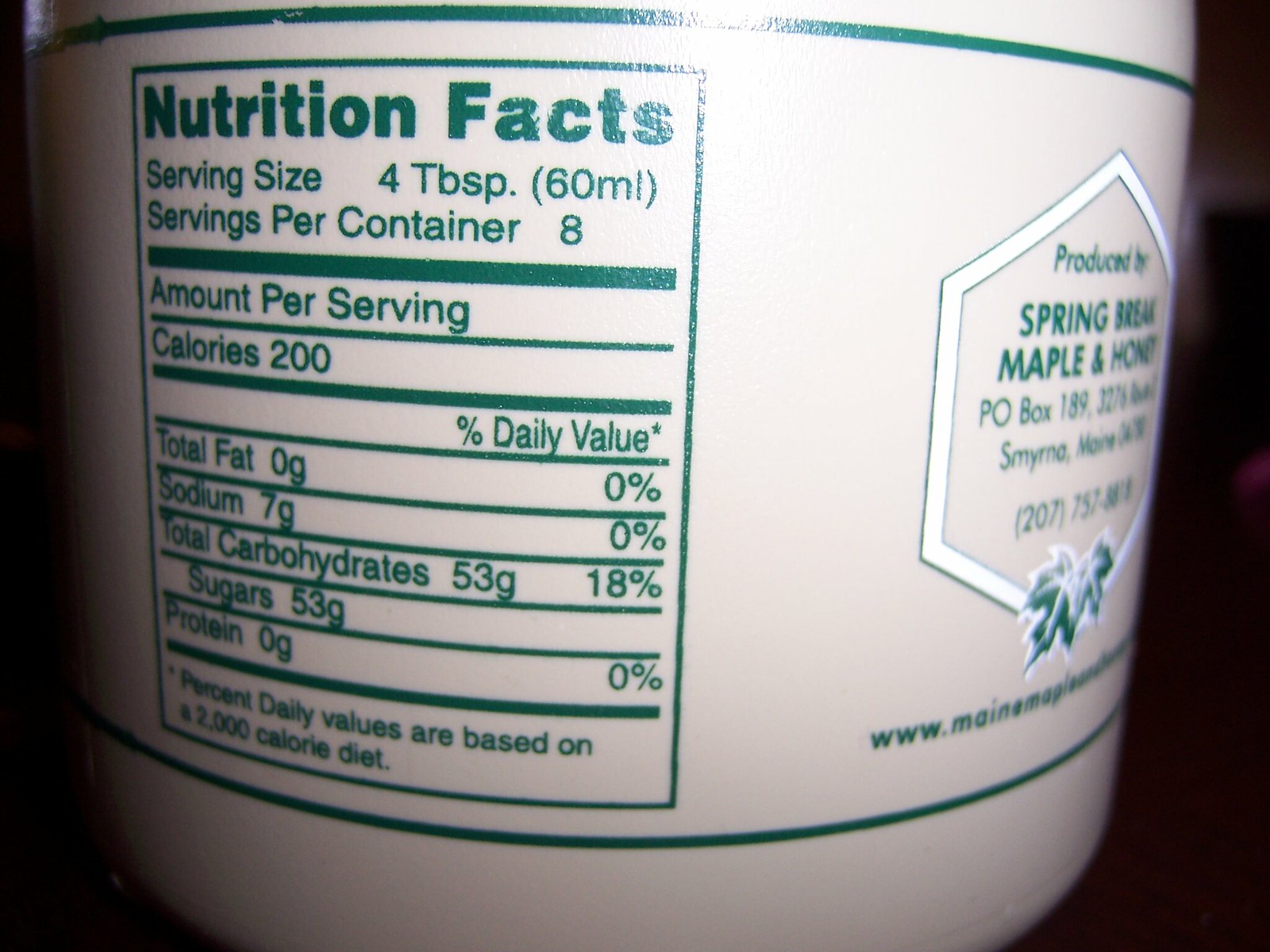In this rectangular image, we see the back label of a food container. The label is predominantly green and contains detailed information about the product. On the right side, it states, "Produced by Spring Break Maple and Honey, P.O. Box 189, Smyrna, New York," in green text. The Nutrition Facts section is prominently displayed in bold green text, listing the following details: Serving Size - 4 tablespoons, Servings per Container - 8. Each serving contains 200 calories, 7 grams of sodium, 0 grams of total fat, 53 grams of total carbohydrates, all of which are sugars, and 0 grams of protein. At the bottom of the label, it reads in smaller green print, "Percent Daily Values are based on a 2000 calorie diet."